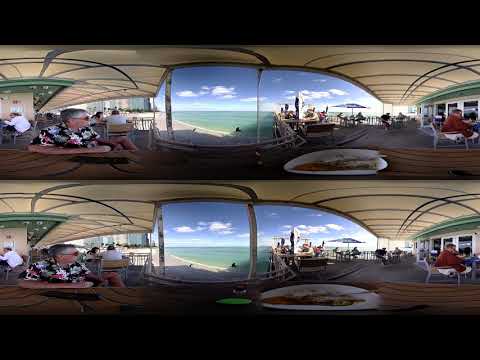The panoramic fisheye photograph depicts an open-air restaurant by the sea, presenting a warped, curved visual of its cozy dining area. The image, replicated identically on the top and bottom of the frame, showcases an inviting setup where several tables and chairs are occupied by patrons. The restaurant boasts a cream-colored roof, sheltering diners from the bright blue sky dotted with white clouds. The open side of the restaurant provides an unobstructed view of the serene blue sea.

On the right side of the image, near the waterline, there's a visible umbrella that appears to be a part of an outdoor seating arrangement. At the forefront, a diner in a black or navy blue shirt with white fluorescent patterns is discernible, seated at a brown table, partly consumed by their meal on a white plate. Another patron, clad in a red jacket, is seated nearby, adding to the lively ambience.

In the midst of the scene, wooden structures support the central awning, creating a rhythm of curved black and cream-colored lines that repeat in the mirrored bottom half. The left side of the image features a man's face in profile, sporting sunglasses, which is echoed in both the upper and lower halves of the composition.

Together, these elements create a dynamic, immersive visual experience, illustrating the convivial atmosphere of seaside dining and the detailed curvature brought by the fisheye lens.